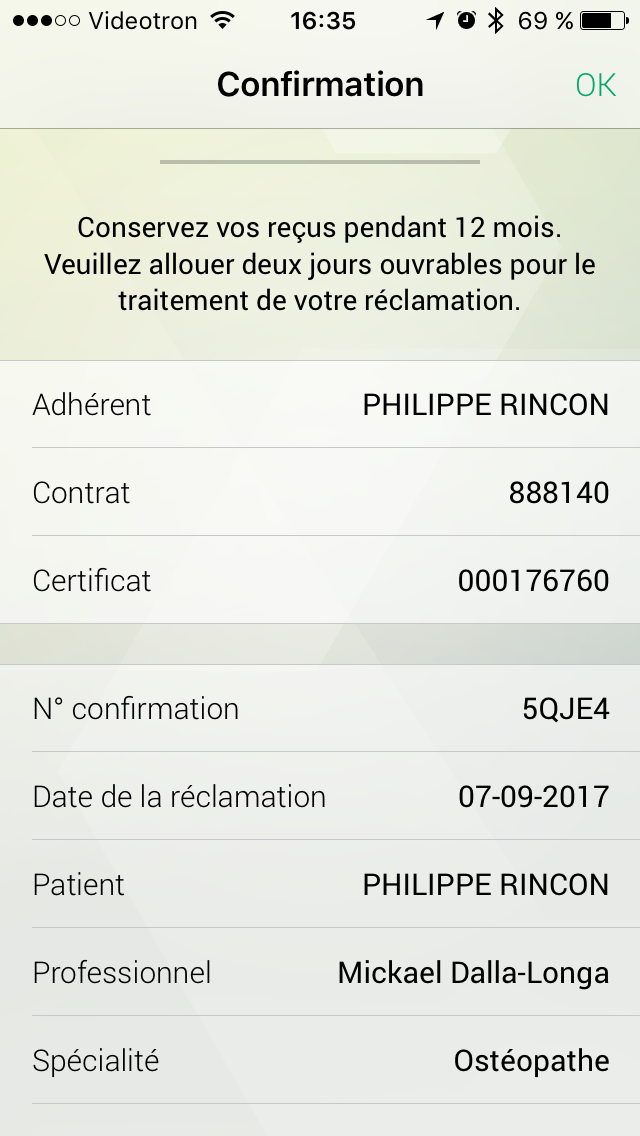The screenshot from a phone displays a confirmation screen with "Videotron 1635" at the top, indicating the time as 16:35 and a battery level of 69%. Below, in black letters, the word "confirmation" is prominently displayed, along with a green "OK" button to the right. The text beneath is a paragraph written in French, followed by a detailed list of information in two horizontal columns. Notable entries include Michael Dallalonga, indicating his specialty as an osteopath, and another name, Felipe Rincon. Additional rows contain various details such as contract numbers like 888144 and certificate numbers like 000176760. There is also a date, 07/09/2017, possibly marking the confirmation date. The background colors vary from white to tan and there are several bolded items on the right column of the list, which organize various pieces of information systematically.